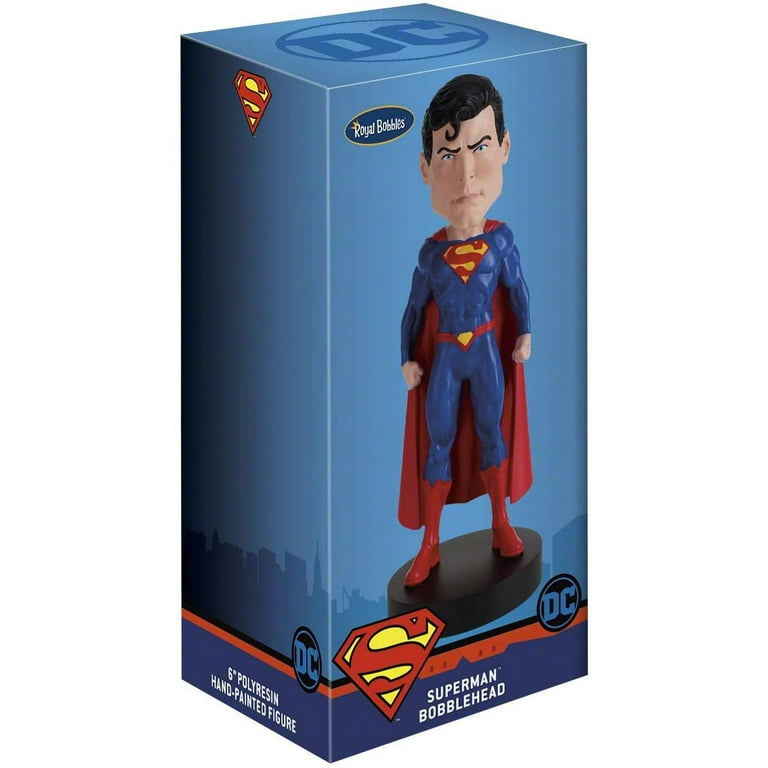The box is a rectangular, tall packaging with a light blue gradient background, prominently featuring a Superman bobblehead figure. The top of the box displays a circle with the DC logo in large letters. The brand "Royal Bobbles" is present in a blue oval with a yellow border, located at the top left corner. The front of the box shows a detailed Superman figure dressed in a blue spandex suit, complemented by a red cape, red boots, red belt, and a distinctive yellow and red "S" triangle on his chest. Superman has black hair styled with a signature curl over his forehead, reminiscent of the classic Christopher Reeves portrayal. His stance is dynamic, with one fist clenched.

In addition, the figure's description on the packaging reads "6 inch polyresin hand painted figure" in white text. The bottom of the box also displays the Superman logo prominently. On the left and right sides of the box, the DC logo appears again, along with the Superman emblem. The bottom right corner of the front side has a combined black and blue DC Comics logo. A city skyline silhouette adorns the lower section of the side panels, emphasizing the superhero’s connection to Metropolis. Overall, the box emphasizes the officially licensed and collectible nature of the Superman bobblehead.